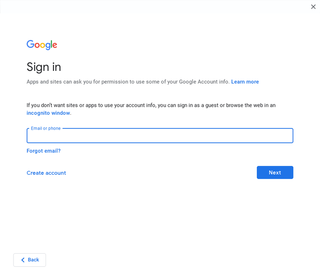The image displays a Google sign-in page.

In the top-left corner, the prominent multicolored Google logo is visible, showcasing the letters "G" in blue, "o" in red, "o" in yellow, "g" in blue, "l" in green, and "e" in red. Below the logo, in a blackboard-style font, is the text "Sign in" with an emphasized capital "S." Directly beneath this, there is smaller black text stating: "Apps and sites can ask you for permission to use some of your Google Account info." Following this statement, a clickable "Learn more" link is highlighted in blue.

In the top-right corner of the page, there's a dark gray "X" icon that allows users to exit the screen. Beneath the smaller introductory text, there is another informative message in black that reads: "If you don't want sites or apps to use your account info, you can sign in as a guest or browse the web in an incognito window." The phrases "sign in as a guest" and "incognito window" are clickable and displayed in blue text.

The central feature of the page is an editable field designed for user input; it is a long rectangular box with a blue outline. The outline is slightly rounded at the corners and has a break at the top left where it states "Email or phone" in blue text. This field is where users can enter their credentials. Below this input space, a blue "Forgot email?" link is available for those who may have forgotten their login details.

Towards the bottom right of the input box, there is a dark blue, filled rectangular button with the word "Next" written in white, indicating the next step in the sign-in process. To the left of this button is a "Create account" link in blue text for new users wishing to register. In the bottom left corner, there's a "Back" button also in blue, allowing users to return to the previous page.